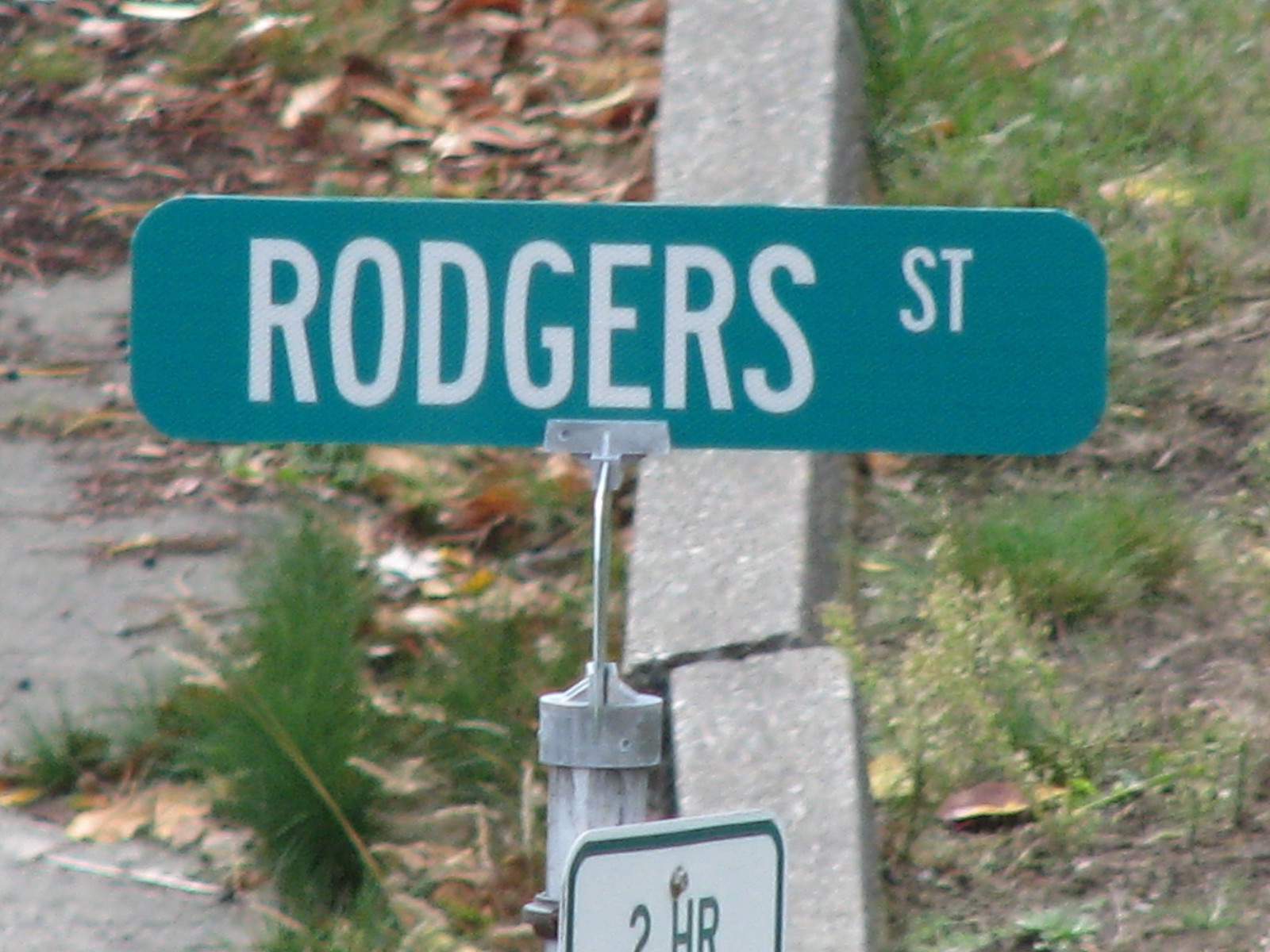This outdoor photograph, taken on an overcast day, showcases a horizontal landscape-style image focusing on a street sign. The sign, labeled "ROGERS ST," is a typical green street sign with large white capital letters for "ROGERS" and smaller letters for "ST." It is mounted on a worn, silver metal pole that stretches down to the bottom of the image. Beneath it, a white rectangular parking sign with a green border is bolted to the same pole, and it reads "TWO HOUR."

The background of the image features two cement rectangular slabs running vertically, separating a patch of green grass and dirt on the right from a road on the left. Scattered across the dry, brown earth next to the curb, which is cracked and slightly misaligned, are piles of wet, brown leaves and twigs, indicative of colder weather. The ground looks dry with some sparse greenery such as weeds, and the scene is divided by cylinder blocks likely segregating the parking areas.